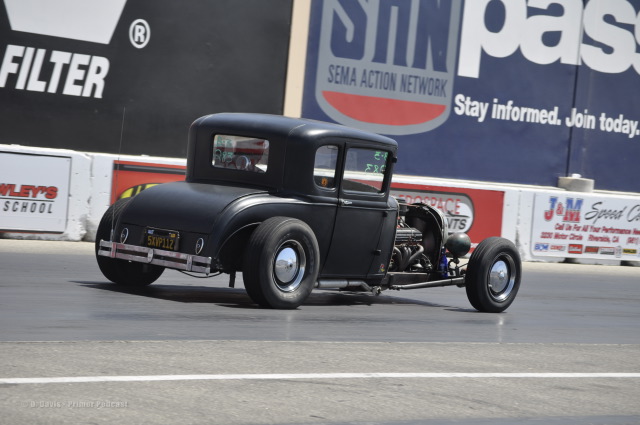The photograph captures a black, vintage car, reminiscent of styles from the early 20th century to the 1960s, racing on a gray racetrack marked with a white line. The car's front panels are removed, exposing its engine, and it features a covered roof. The image provides a side view of the car, which appears to be in motion. Surrounding the track are numerous banners and advertisements, with some being identifiable: a black sign with "FILTER" in white letters, and a blue sign bearing the message "SEMI ACTION NETWORK, STAY INFORMED, JOIN TODAY" with partially visible letters "P.A.S." The advertisements vary in color, including red, white, blue, and black. The concrete edges of the track and the multitude of vibrant ads create a dynamic, nostalgic racing scene.